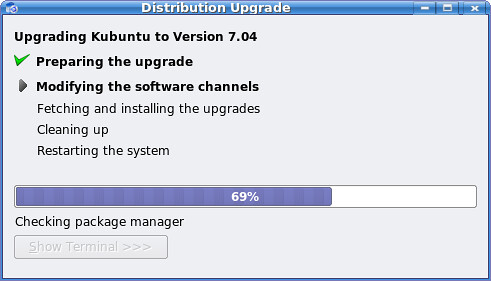The image depicts a screenshot of a computer monitor displaying the status of an ongoing distribution upgrade. At the top of the window, there's a blue taskbar featuring standard window control buttons: an X to close, an arrow for full screen, and a minus sign to minimize. In white text within this blue bar, it reads "Distribution Upgrade." Below the taskbar, the background of the window is grayish light blue, and in dark black text, it states "Upgrading Kubuntu to version 7.04." A green check mark is placed next to "Preparing the upgrade." Under this, a dark arrow points to "Modifying the software channels," indicating the current step in the process. Further listed steps include "Fetching and installing the upgrades," "Cleaning up," and "Restarting the system." A blue progress bar at the bottom shows that the upgrade is 69% complete, transitioning from blue to white to signify progress. Additionally, beneath the progress bar, there is text indicating "Checking package manager" and a button labeled "Show Terminal."